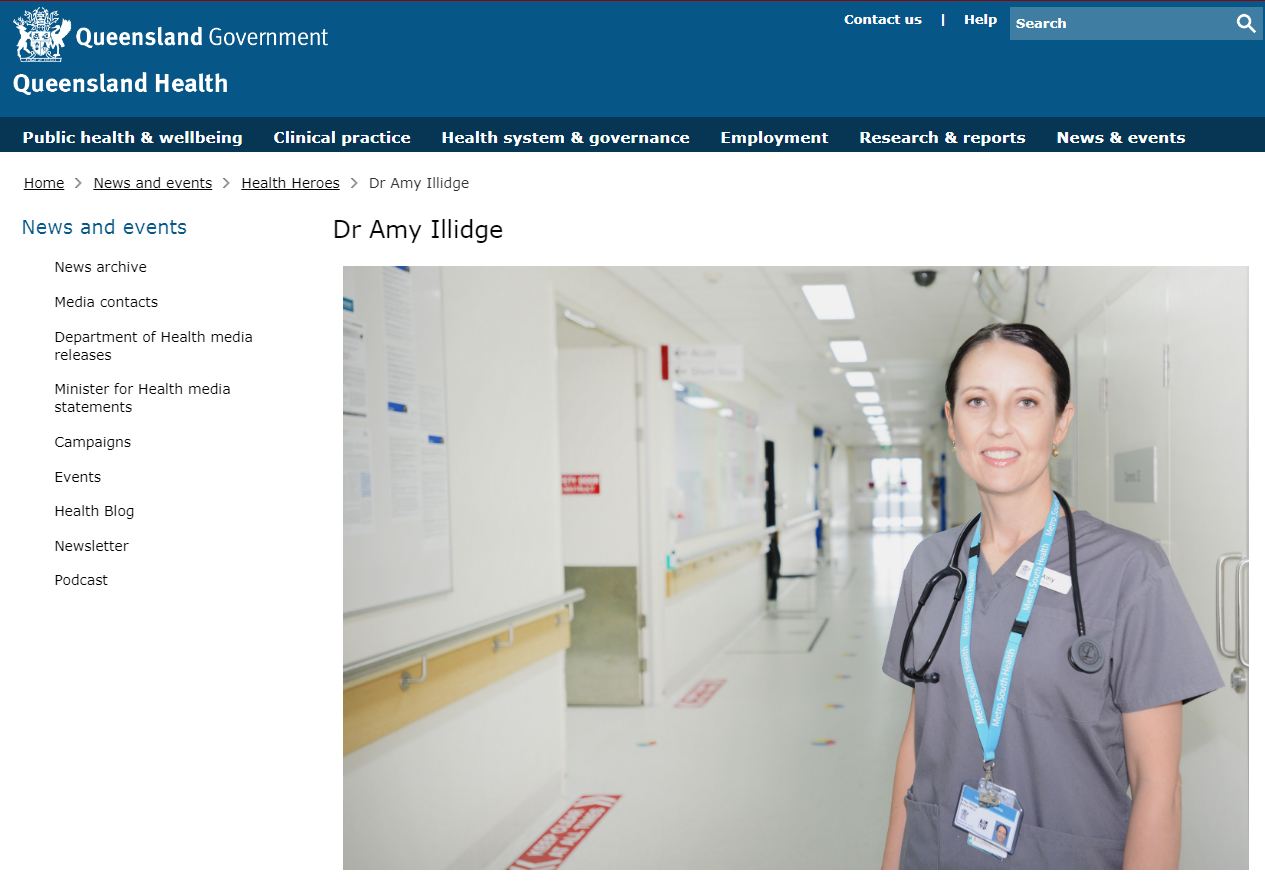This image, sourced from the Queensland Government website, features a detailed layout typical of a public health webpage. To the right of a prominent blue border is a contact help icon and a search box. Directly below is the Queensland Health logo on the left. Following this section, in a darker blue, there are navigation tabs labeled "Public Health and Well-being," "Clinical Practice," "Health System and Governance," "Employment," "Research and Reports," and "News and Events."

Beneath this, in a white area which comprises the main body of the page, there are additional tabs including "Home," "News and Events," "Health Heroes," and a highlighted "Dr. Amy Hilditch." This section features a photograph of Dr. Amy Hilditch, a European-descended woman in her 30s, standing in the pristine, white hallway of a hospital or clinic. She is dressed in medical scrubs with a stethoscope and an ID badge around her neck, and her hair is neatly pulled back.

To the left of Dr. Hilditch's photograph, there are subsections labeled "News and Events," "News Archive," "Media Contacts," "Department of Health Media Releases," "Minister for Health Media Statements," "Campaigns," "Events," "Health Wall Newsletter," and "Podcast."

The hallway in which Dr. Hilditch is standing is immaculately white, reflecting cleanliness and a sterile environment. Overhead, fluorescent lights run the length of the hallway, enhancing the bright, sanitized appearance of the space.